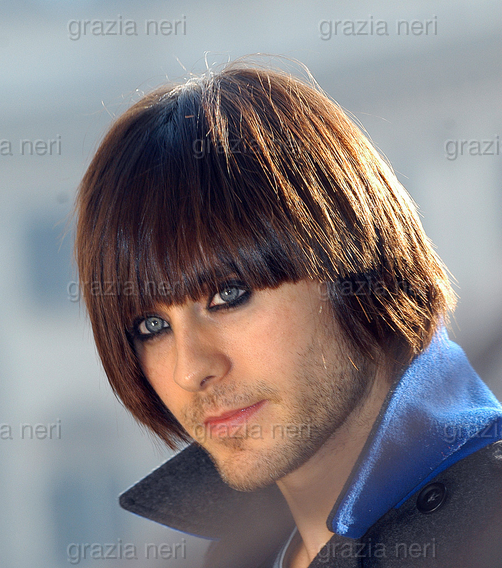The image is a professional photograph featuring Jared Leto, an actor and singer, prominently positioned in the center against a blurred, grayish-white background. The background is patterned with the watermark "Grazia Neri" repeatedly printed in various lines, creating a texture without clear definition. Jared Leto is looking slightly off to his left, with his head turned subtly towards the viewer. He sports a distinctive, androgynous look with a bob hairstyle that has bangs falling just past his eyebrows, long hair that reaches his chin and covers his ears, and strong mascara accentuating his bright blue eyes. He has a stubble beard adding to his masculine-feminine aesthetic. Jared is dressed in a stylish gray coat with a dark button on the left shoulder of the collar, which is notably blue on the outside and gray on the inside. Underneath the coat, he wears a silky blue shirt with the collar slightly sticking up on his left side. The composition, coloring, and style of the photograph emphasize a sophisticated yet edgy look, attributed to Grazia Neri.